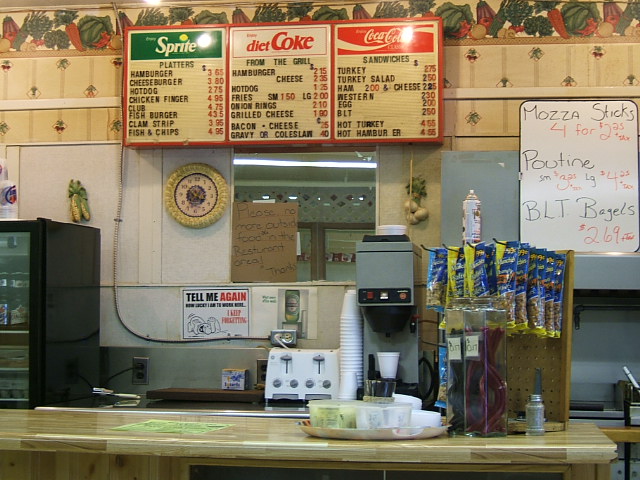This photograph captures a bustling segment of a restaurant's counter area. The counter, designed for patrons to sit and enjoy their meals, showcases part of the back and front-end operations. Prominently featured in the background is a large, red-framed menu display advertising popular beverages like Sprite, Diet Coke, and Coca-Cola. Below this are manually adjustable letter slots, indicating today's offerings which include platters from the grill, sandwiches, and miscellaneous items.

A whiteboard also makes an appearance, listing special items such as mozzarella sticks, poutine, and BLT bagels. Clearly visible on the back counter are kitchen essentials like the edge of a stove or grill and what seems to be a toaster. On the left side of the image, a cooler stocked with beer bottles can be seen.

The customer-facing counter displays an array of goods as well. In one corner, there's a small display area showcasing bagged peanuts and other items for sale. The counter itself is made of blonde wood and holds a greenish menu. Additionally, a mirror mounted on the wall has a cardboard sign taped to it, reading, "Please no outside food in restaurant area, thanks."

This detailed setup paints a clear picture of the vibrant and functional dining and service area within the restaurant.